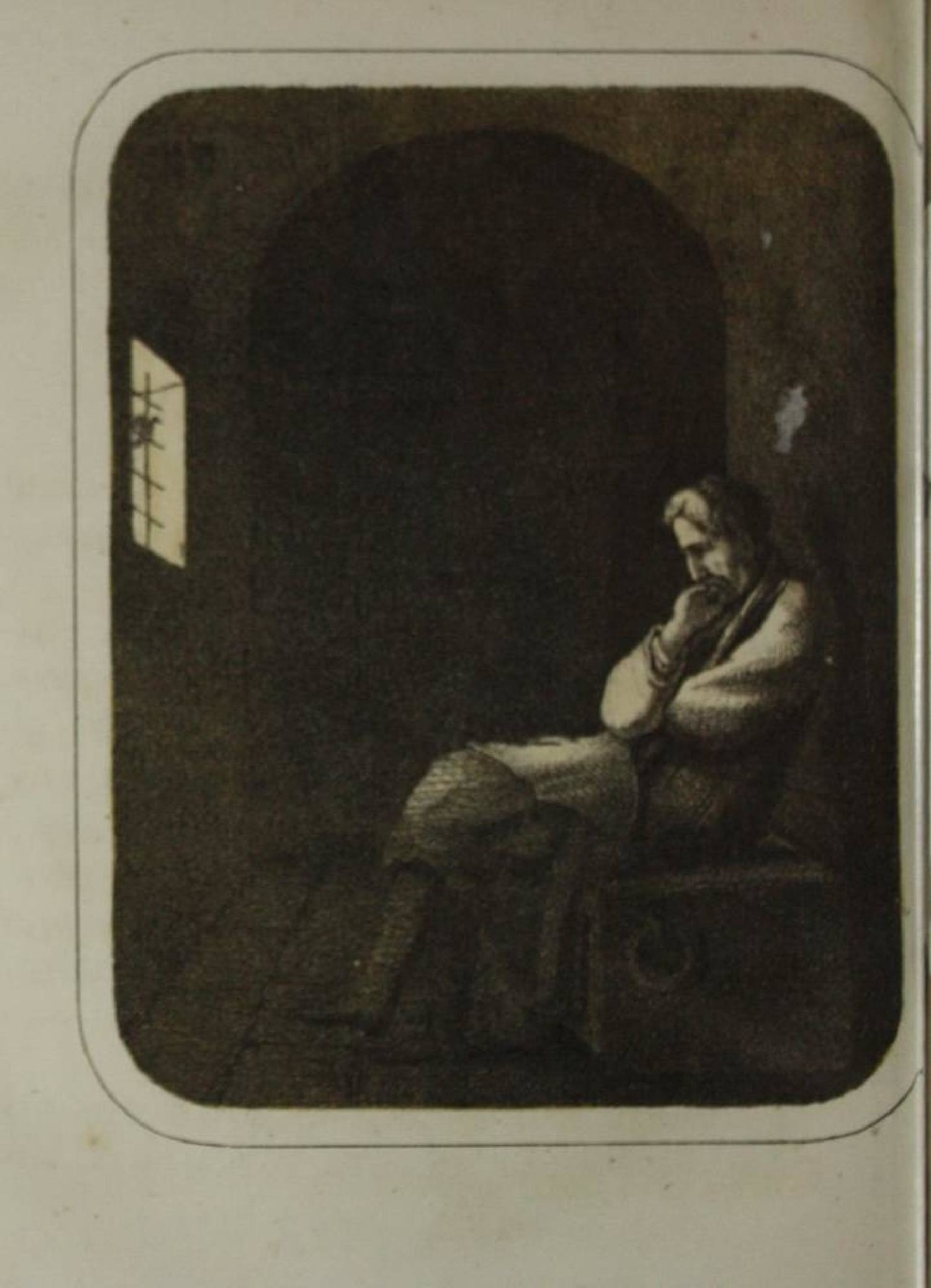The image is a black and white photograph of a drawing, rendered on white paper without a signature or date. The background of the drawing is predominantly black, featuring the silhouette of an arched doorway that suggests a hallway extending from the scene. To the left, a window emits bright sunlight, casting reflections onto the wall behind a solitary man seated in a decorative chair with a spiraling design underneath. The man's long hair is parted in the middle, and he has a beard and mustache. His posture is thoughtful, slouched slightly with his right leg crossed over his left. He holds his left forearm with his right hand, his left hand propping his chin in a pensive manner. The contrast between the illuminated parts of his face and body against the darker surroundings emphasizes his contemplative state, while the stone floor and sparse furnishings evoke the atmosphere of a monastery.